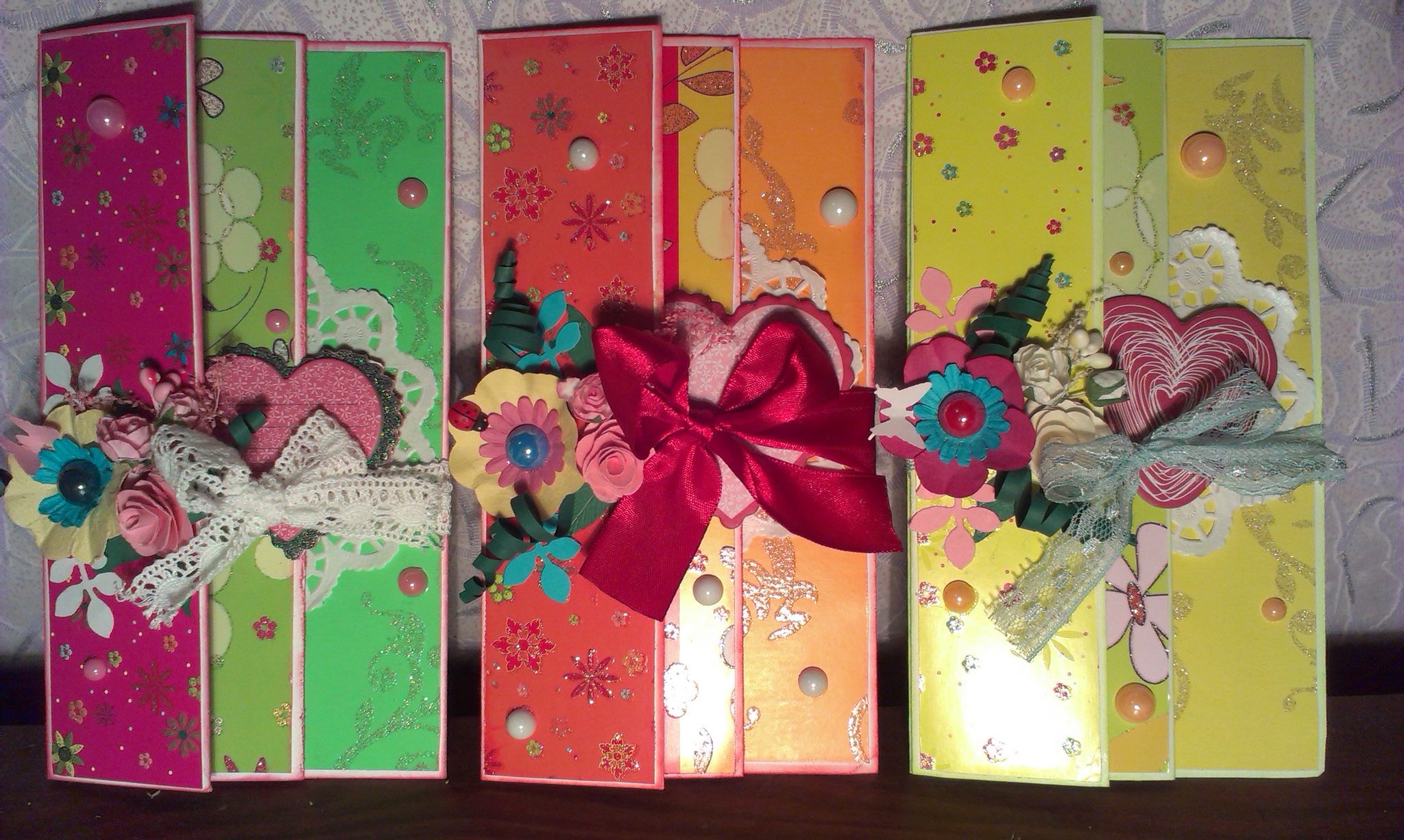The image is a vibrant color photograph taken in landscape orientation, depicting three intricately decorated cards that stand vertically on a dark wooden table. These cards, seemingly handmade and of high quality, are folded pieces of cardboard, each distinct in its color scheme and adorned with unique embellishments.

The first card on the left features panels with shades of pink, light green, and dark green, each adorned with floral designs. It is tied together with a white lace ribbon, creating a bow that secures the card's flaps. The ribbon also has paper flowers attached, enhancing its delicate appearance.

The middle card showcases a palette of reds and oranges, with intricate snowflake patterns and glittery embellishments in red and green hues. This card is fastened in the center with a fuchsia or pink satin bow, further complemented by 3D paper flowers and fake pearls, giving it a festive look.

The rightmost card predominantly uses greens, yellows, and lime green colors, with panels varying from a light greenish-yellow to darker shades of yellow with glittery flower designs. A light blue lace ribbon ties this card, finished with cut-out paper flowers and leaf motifs.

Set against a background of light grayish-white floral designed wallpaper, the photograph captures the intricate details and vivid colors of these standing cards, each with its unique decorative elements and cohesive design.